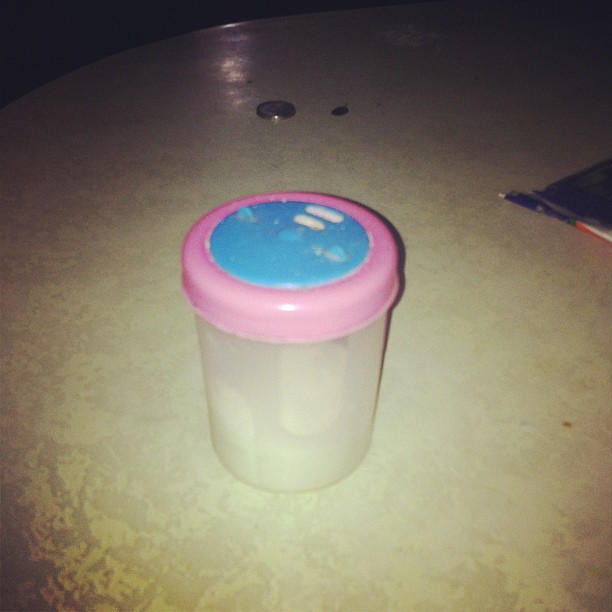The image features a transparent pot with a pink and light blue lid, situated on a circular table. The pot is designed with two holes in the lid, making it appropriate for containing powdery substances like salt or flour, though it appears to be empty. To the right of the pot lies a blue pencil, and further back in the image, a notebook slightly intrudes from the upper right corner, with a black and red pen attached to it. In the background, there is a small silver object, possibly a penny, resting in the shadows. The scene is illuminated by a camera flash, casting light reflections on the table and creating dark, night-like surroundings.